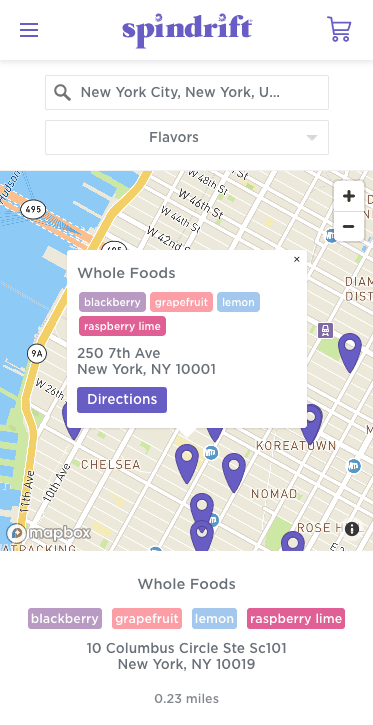**Caption:**

A detailed screenshot of a map application interface. At the top, a purple banner features the word "Spindrift." Directly beneath is a search bar displaying "New York City, New York." Below this, the section titled "Flavors" appears. The main map area shows a pop-up box identifying a location named "Whole Foods." The pop-up includes various tags indicating flavors: blackberry, grapefruit, lemon, and raspberry lime. The specific address given is 257th Avenue, New York, NY 10001. At the bottom of the pop-up box is a purple "Directions" button for navigation assistance.